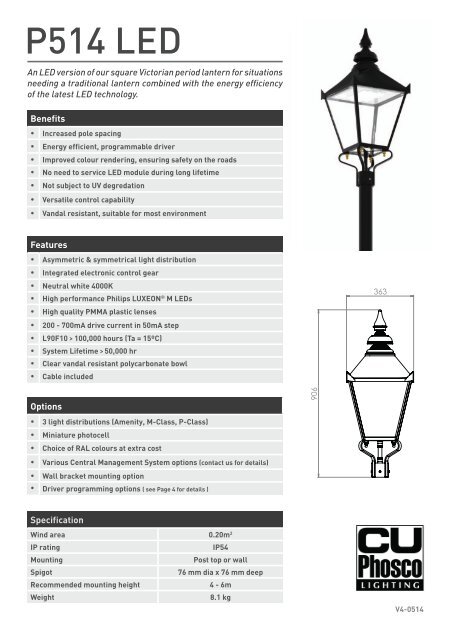This is an elaborate advertisement or options page for a LED version of an outdoor lantern, labeled prominently as "P514 LED" in uppercase black text against a white background.

---

**Product Description:**

An LED iteration of our square Victorian period lantern, ideal for settings that demand a traditional aesthetic while benefiting from the energy efficiency afforded by modern LED technology.

---

**Benefits:**

- **Increased Pole Spacing**: Enhances the overall lighting coverage area.
- **Energy Efficient**: Reduces energy consumption.
- **Programmable Driver**: Allows for customized lighting settings.
- **Improved Color Rendering**: Delivers superior light quality.
- **Ensuring Safety on the Roads**: Provides consistent and reliable illumination.
- **Long Lifetime**: Minimal need for servicing the LED module.
- **UV Degradation Resistant**: Maintains quality and performance over time.
- **Versatile Control Capability**: Adapts to various control systems.
- **Vandal Resistant**: Built to withstand tampering and damage.
- **Suitable for Most Environments**: Versatile usage across different settings.

---

**Features:**

- **Light Distribution Options**: Available in asymmetric and symmetrical configurations.
- **Integrated Electronic Control Gear**: Ensures efficient operation.
- **Neutral White Light**: 4000K color temperature for optimal lighting.
- **Philips Luxion M LEDs**: High-performance LED technology.
- **High-Quality PMMA Plastic Lenses**: Durable and efficient light diffusion.
- **Drive Current**: Configurable from 200 to 400 mA in 50 mA steps.
- **L90F10 > 100,000 Hours**: Ensures a long operational lifetime.
- **Thermal Management**: 1A equals a 15-degree Celsius temperature.
- **System Lifetime**: Greater than 50,000 hours.
- **Clear Vandal Resistant Polycarbonate Bowl**: Provides a protective outer layer.
- **Cable Included**: Ready for installation.

---

**Options:**

- **Light Distribution Configurations**: Three distinct options available—amenity M, class P.
- **Miniature Photocell**: Optional feature for automated lighting control.
- **RAL Color Choices**: Custom colors available at an additional cost.
- **Central Management System Options**: Various systems available, contact for details.
- **Wall Bracket Mounted Option**: Additional driver programming options, see page 4 for details.

---

**Specifications:**

- **Wind Area**: (Detailed wind area specifications)
- **IP Rating**: (Ingress Protection rating)
- **Mounting and Spigot**: (Details on mounting methods and spigot size)
- **Recommended Mounting Height**: (Optimal height for installation)
- **Weight**: (Product weight information)

---

**Diagrams:**

- **Top View of the Lantern**: Detailed top-angle diagram.
- **Size Specifications**: Middle section shows size dimensions.
- **CU Phosco Lighting Version 40514**: Detailed specifications of the lighting version.

**Contact Information:**

For more details on customization and options, contact CU Phosco Lighting.